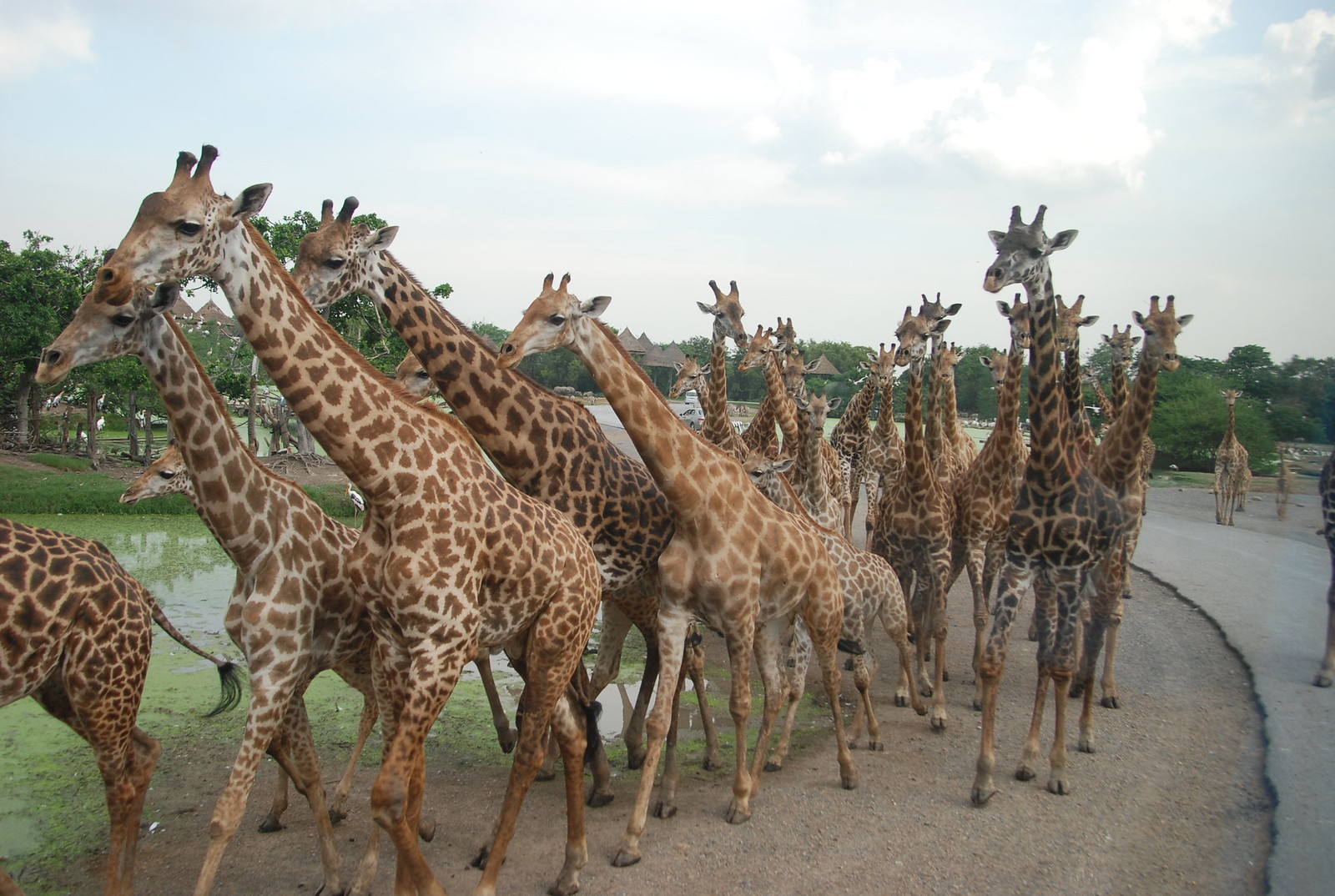In this detailed photograph, you can see a sizable herd of approximately twenty giraffes walking along a curved pavement, positioned primarily in the center and left of the frame with a few stragglers to the right. The giraffes are patterned in white and orangish-brown spots, with no text present in the image. The scene is set outdoors under a light blue sky dotted with white clouds. The background features a series of full, bright green trees, with some darker green hues interspersed. To the left of the foreground, there's a body of water topped with algae. Alongside the pavement and to the right of the giraffes, there are what appears to be poles with brown canopies, resembling small huts or shelters. This vivid image captures the essence of a natural habitat, potentially within a zoo, showcasing the giraffes walking in harmony along their path.